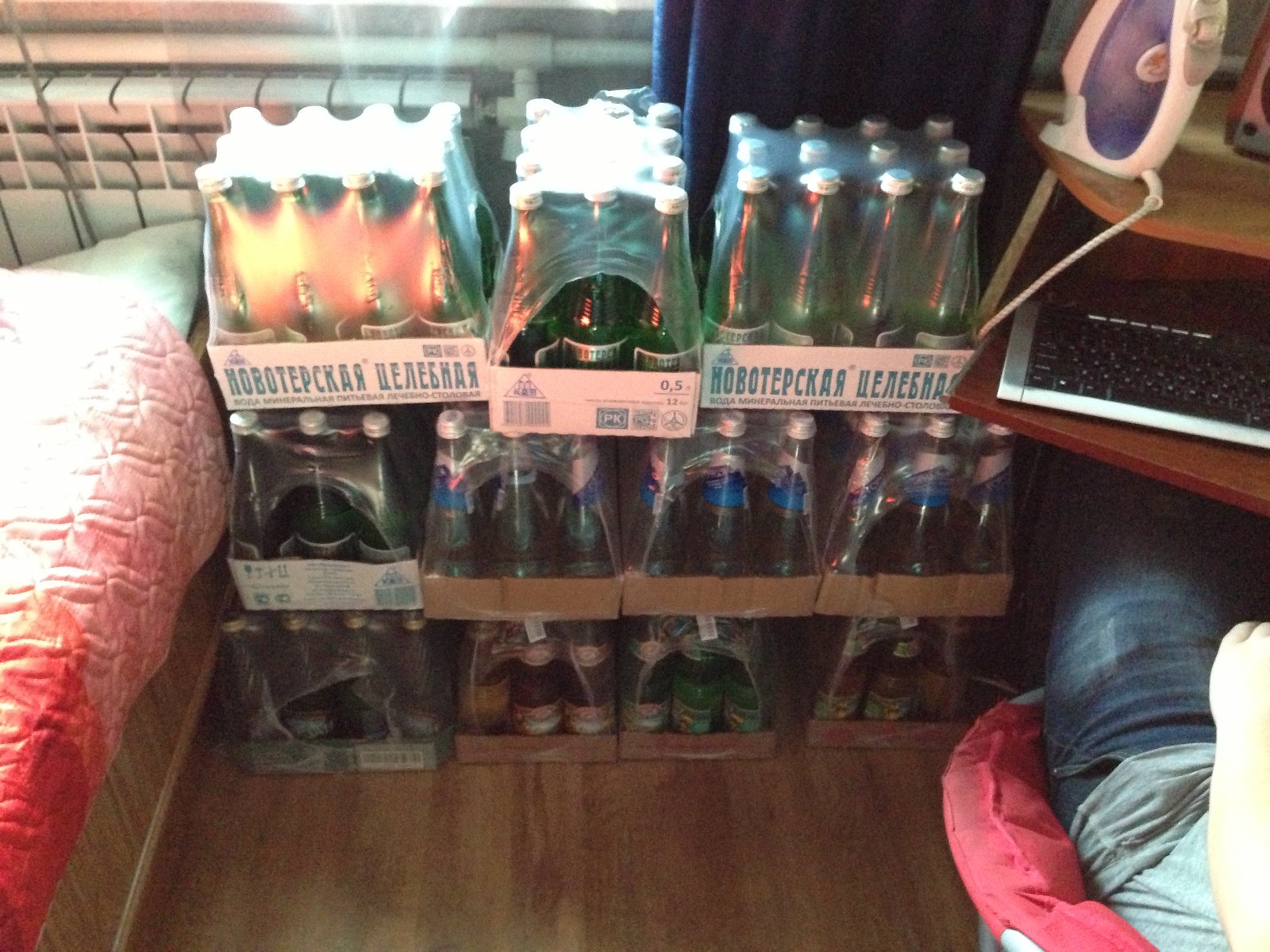The photograph depicts the interior of a room featuring three neatly stacked rows of bottled drinks, each case holding 12 tall glass bottles with white caps. The packaging bears writing in Russian. The bottles exhibit a variety of colors, including green, red, and possibly dark blue or black, suggesting different flavors or types of drinks. In the bottom right corner, a person is seated on a comfortable pink chair, identifiable by their blue denim jeans, gray t-shirt, and extended left hand. To the left, there is a bed with a pink and red comforter. In the top right corner, a computer desk is visible, equipped with a keyboard and an old desktop speaker.